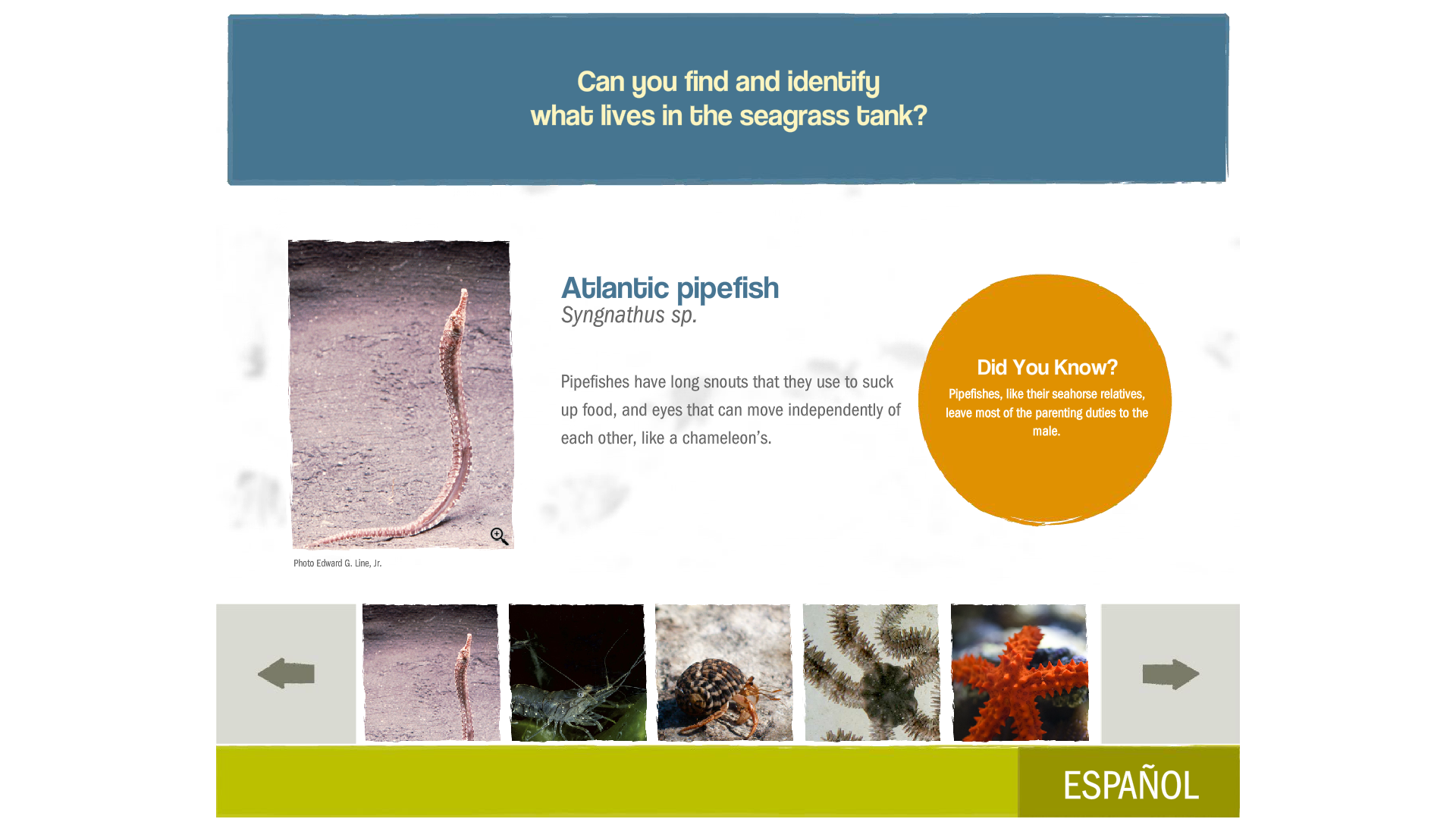The image appears to be a screenshot of an educational app with detailed information about marine life. 

At the top, there is a prominent blue bar with a slightly faint yellow text that reads: "Can you find and identify what lives in the seagrass tank?"

Beneath this bar, on the left, there is an image of a fish, speculated to be a notable species within marine biology. Directly underneath the fish image, there's some small text that is unreadable. To the right of the fish image, in larger, blue text, the caption identifies the species as "Atlantic Pipefish." Below this, the scientific name of the pipefish is presented in italicized black text. 

Further below, detailed information about the Atlantic Pipefish is provided in smaller black text: "Pipefishes have long snouts that they use to suck up food, and eyes that can move independently of each other like a chameleon's."

To the right of this description, there is an eye-catching orange circle with a "Did you know?" heading in large text. Below this, in smaller text, it informs the reader: "Pipefishes, like their seahorse relatives, leave most of the parenting duties to the male."

At the bottom of the main section, there is a horizontal bar displaying a series of pictures of various creatures, suggesting that users can click through the images using arrows on the right and left. It showcases five central pictures, likely different marine creatures.

Finally, at the bottom of the screen is a green bar. On the right side of this bar, there's a clickable option labeled "Español," indicating that users can switch the language to Spanish.